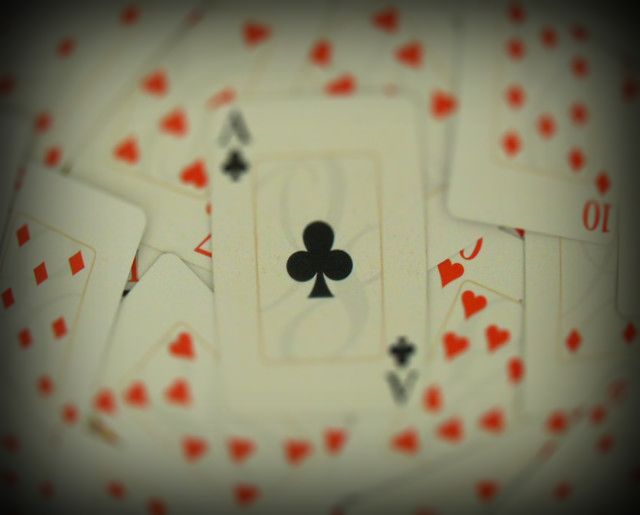This captivating, artistic photograph highlights an ace of clubs playing card prominently positioned at the top of a pile of other cards. Captured with a fisheye lens, the image exhibits the characteristic wide-angle distortion and slightly darkened corners. The ace of clubs card stands out with its white face and a striking black club symbol framed within a brown outline. Surrounding this central card are a mix of red cards, including hearts and diamonds, but their numbers are mostly obscured, contributing to a sense of visual intrigue. The notable exception is a clear ten of diamonds, vividly contrasting against the predominantly red background. This background of red cards is slightly blurred, enhancing the sharp focus on the ace of clubs and creating a dynamic depth-of-field effect. The overall composition and fisheye perspective lend a unique, almost surreal quality to the image.